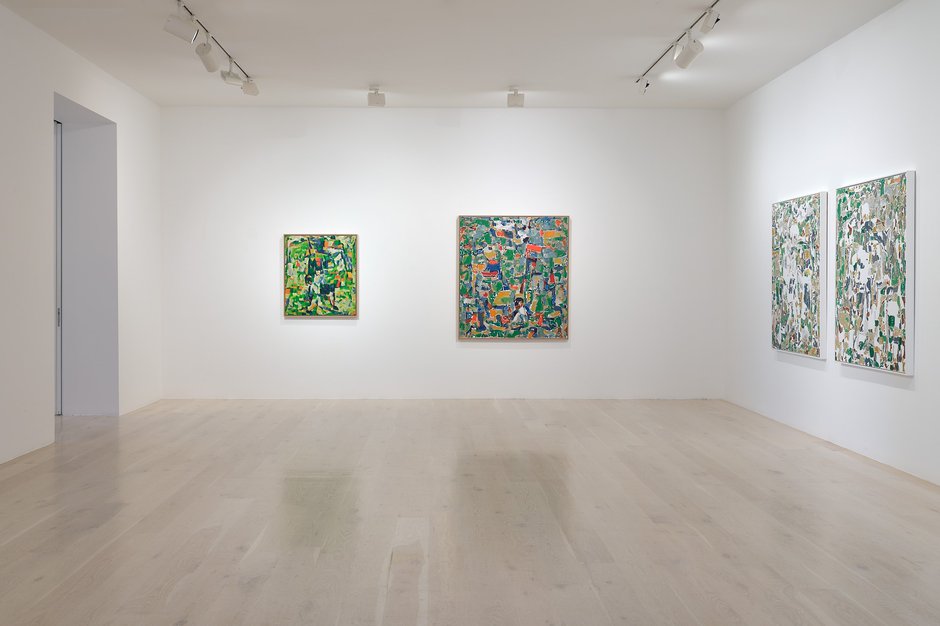This image depicts a spacious and pristine art gallery with white walls and a white ceiling, illuminated by track lighting that highlights the displayed artwork. The floor is polished, light-colored wood, reflecting a sense of cleanliness and elegance. The gallery features abstract artwork that primarily utilizes geometric shapes. Directly in front of the camera, two paintings are displayed on a white wall, with the one on the right being considerably larger. These paintings incorporate a palette dominated by green, along with splashes of red and blue. To the right, there are two other paintings that appear to be a set due to their similar style and muted colors, featuring more whites and light greens. The minimal setup and consistent style of the paintings suggest they could be by the same artist or artists with a cohesive vision. Overall, the room exudes a serene and contemplative atmosphere, ideal for displaying the abstract art pieces.